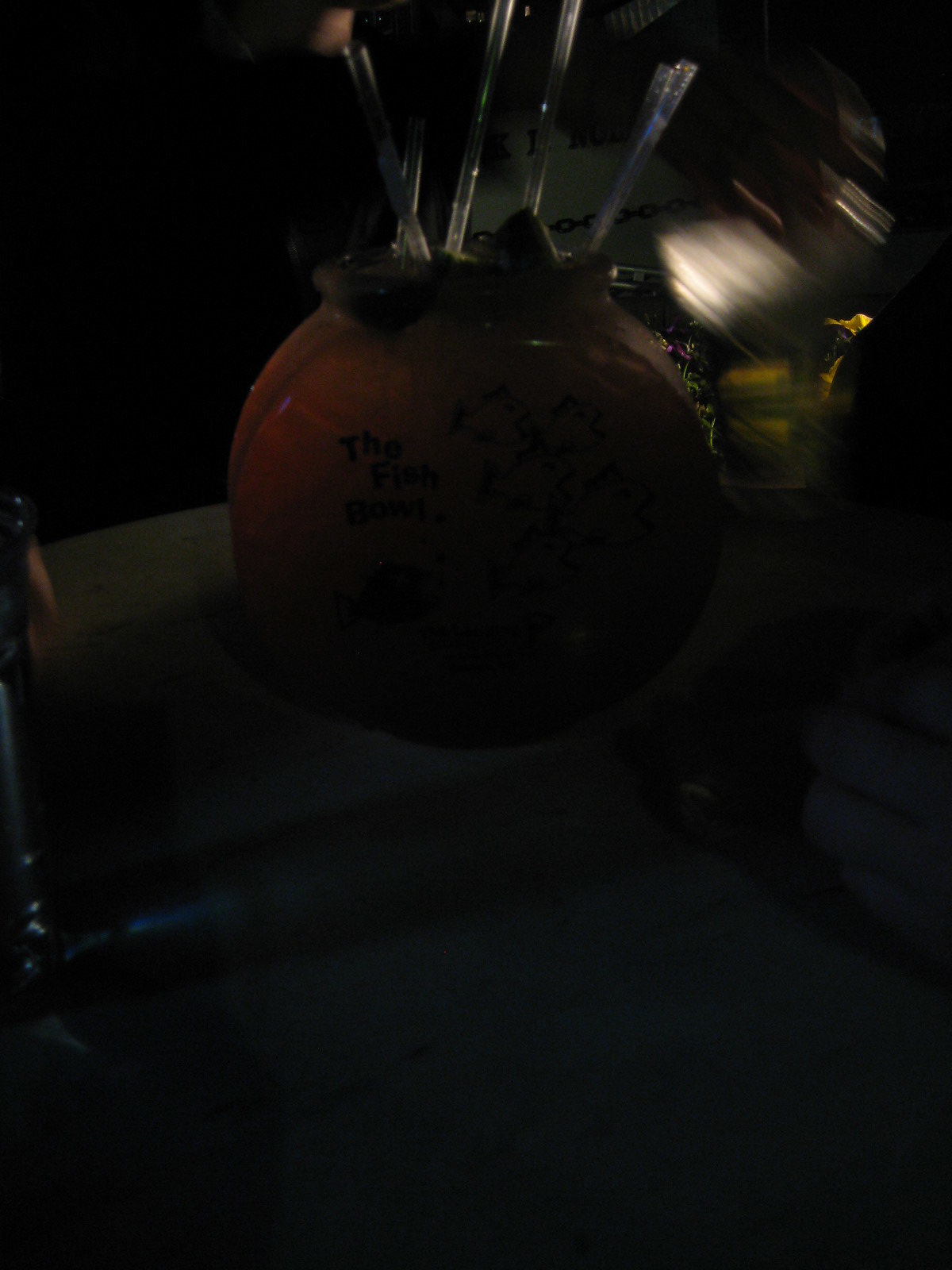The image is a very dark and blurry photograph, making it difficult to discern its contents clearly. At the center, there's a round, brown bowl adorned with black fish drawings and the words "the fish bowl" inscribed on its left side. Protruding from the top of the bowl are five to six transparent straws. To the right of the bowl, there are flowers and a yellow object. Below this, towards the bottom-right corner of the image, a hand holding a black object is visible. A silver object can also be observed on the left side of the bowl. The top portion of the photograph appears to capture some form of light reflection, possibly from aluminum foil or another reflective surface. The dark and indistinct nature of the photograph makes it challenging to identify the finer details.